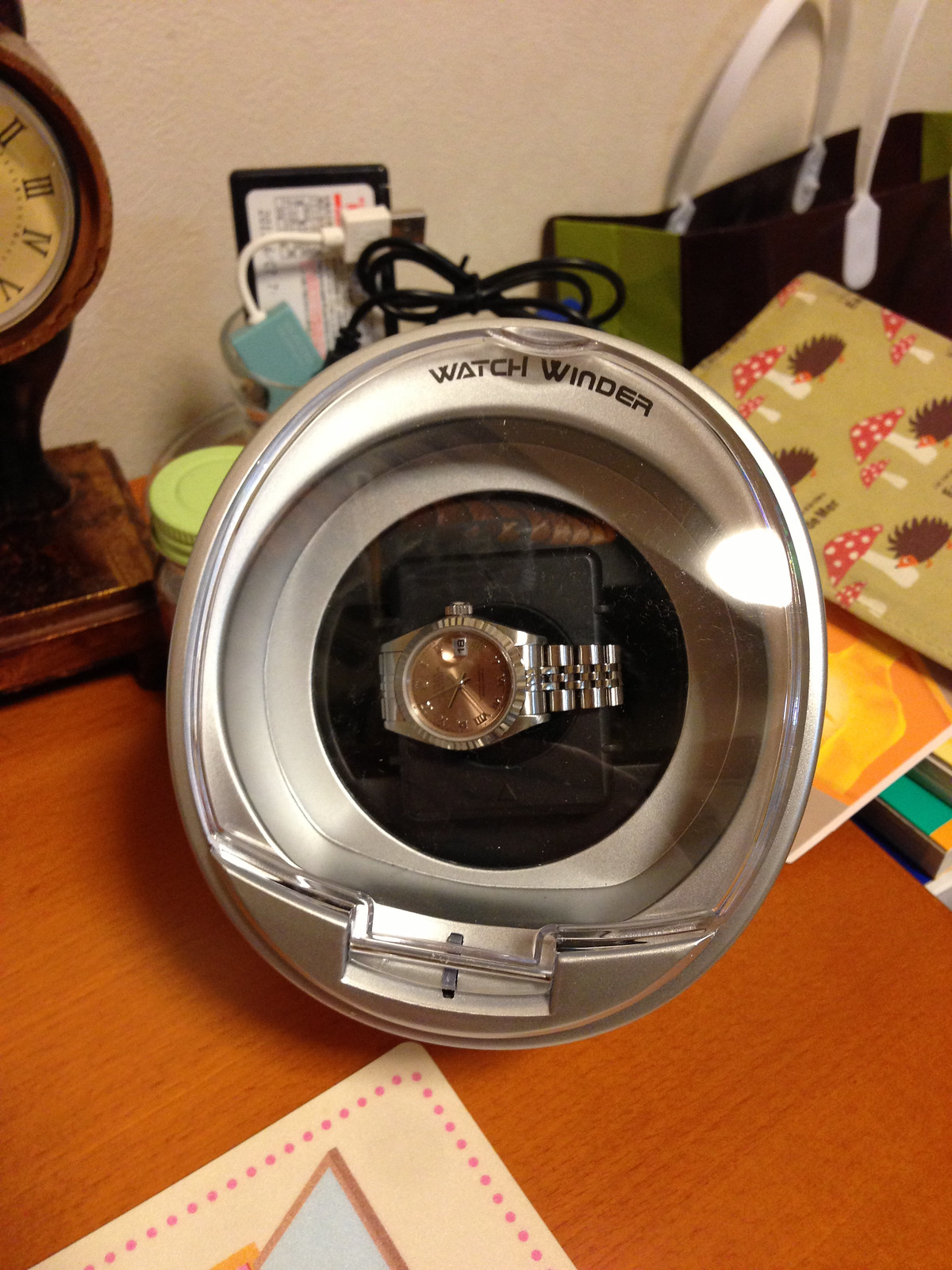In the foreground of the image, there is a watch encased in clear plastic packaging, suggesting it could be a charging station or a holder for the watch when not in use. Behind the watch, there is a small black cable, likely a USB or a DC cable. Also visible is an object encased in clear glass with a USB-A end, possibly a battery pack, featuring a plastic cover with a white label adorned with black and red text, along with some light red, almost pinkish details.

A varnished cherry wood desk forms the base for the setup, upon which a clock with a darker, cherry wood casing and a tan faceplate sits prominently. The clock's face features Roman numerals with additional ticks marking the intervals between them.

To the right of the watch holder, there appears to be a greeting card or possibly multiple cards, adding a decorative element to the scene. Just beyond these cards, there is a gift bag or a shopping bag. In the lower left corner, there is a quarter of another greeting card or possibly a desk accessory peeking into view. The background wall is a light tan or off-white color, contributing to the overall subtle and sophisticated ambiance of the image.